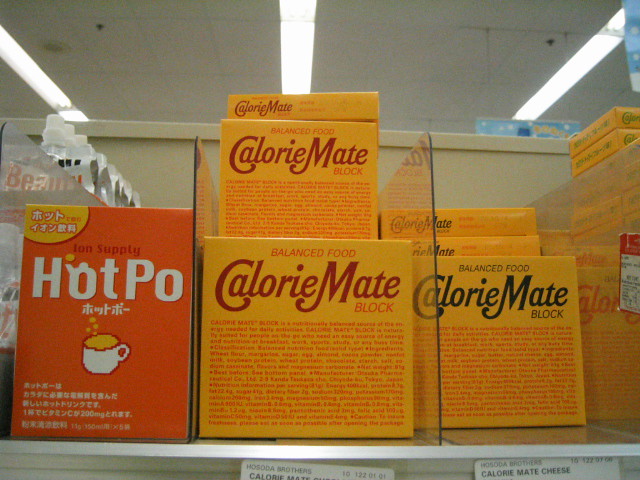The image depicts a store shelf stocked with various products. Prominently featured is "Calorie Mate," a balanced food product packaged in distinct orange boxes. To the left of Calorie Mate, there is "Hot Po," a product encased in a red box, notable for its oriental symbol positioned in the upper left corner. Additionally, a variant of Calorie Mate with different colored font is visible on the right side of the image. Labels on the edge of the shelf below the items indicate that Calorie Mate is recognized as a cheese brand. The shelf holds several units of each product neatly organized. Above, the store's ceiling consists of acoustical tiles and recessed fluorescent lighting, providing a clear view of the stocked items.